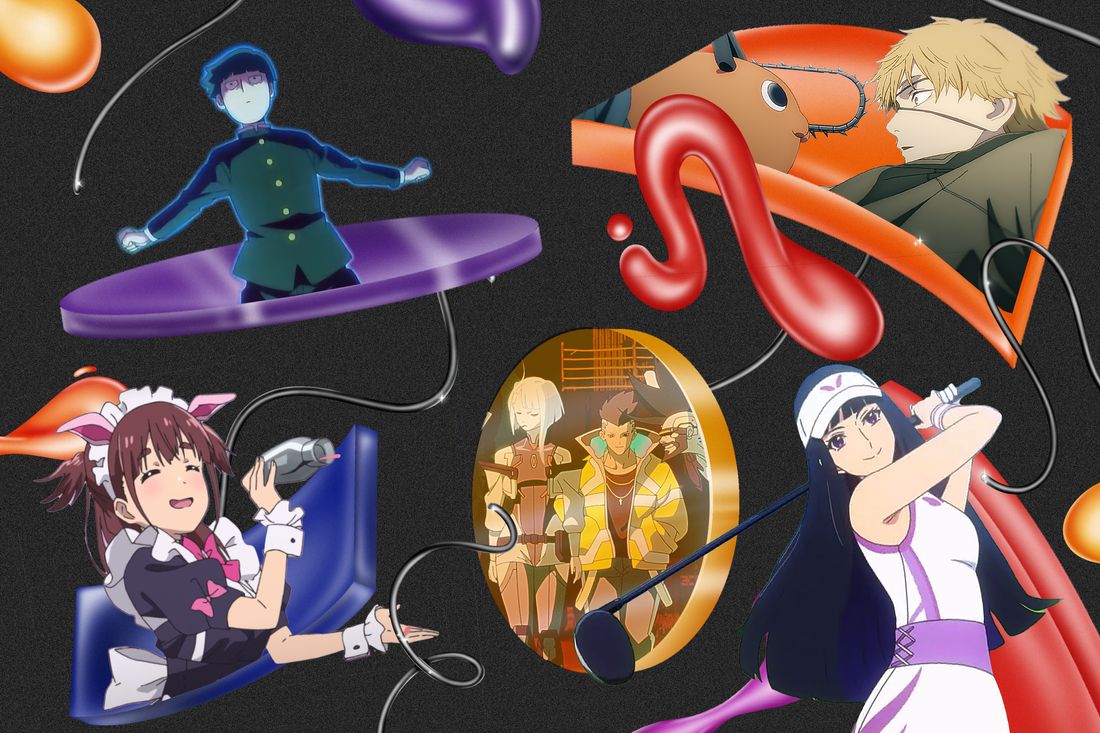The image is a detailed rectangular collage of various Japanese anime characters set against a plain black background, measuring approximately five inches wide and four inches high. In the lower left-hand corner, there is a young female character with light skin, straight brown hair, dressed in a maid's costume adorned with pink bows and pink pig ears, and she’s holding a gray mixing bottle. Towards the center-right, there's an oval containing three characters: a short-cropped white-haired woman, a man with a brown mohawk, and the head of another man with a large, spiked dark brown mohawk and a beard. In the lower right-hand corner, a woman with long black hair is depicted swinging a black-handled golf club; she is wearing a white and purple uniform complete with a visor hat. Above her, a blonde-haired man with an eyepatch is shown gazing at a little creature with a chainsaw for a nose. To the left, a man with black hair, dressed in a black uniform, is kneeling on a purple disc. The top center of the collage features a character with short hair and a green jacket with gold buttons, surrounded by a mix of balloons and squiggly lines, including an orange balloon in the upper left and a purple balloon at the top center. The entire collage has a black, static-like background, uniting all the elements into a cohesive yet dynamic scene.